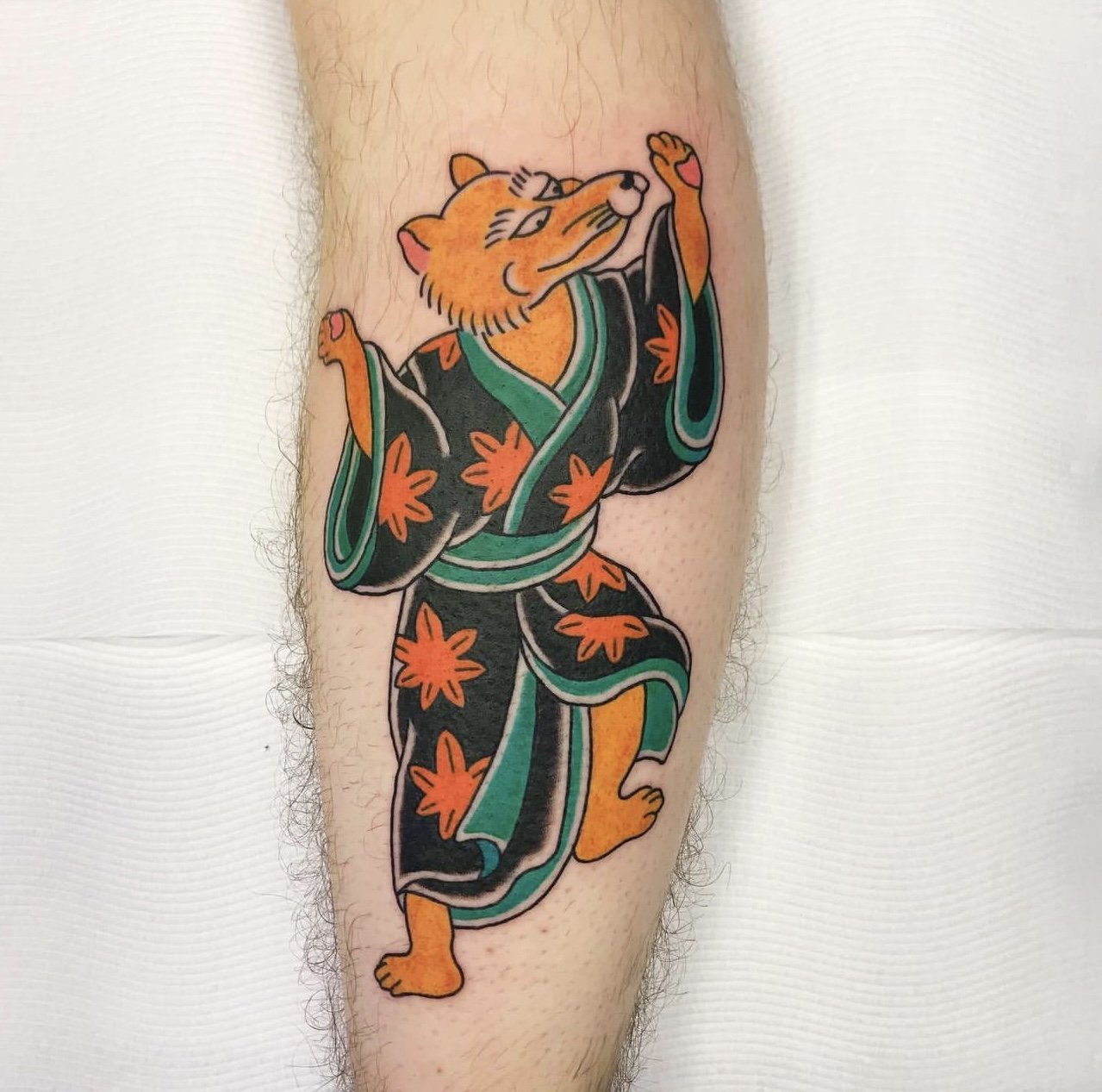The image features a detailed tattoo on the forearm of a Caucasian man, which rests on white paper towels with visible fold marks and a weave pattern. The tattoo depicts a fox-like creature, often mistaken for a coyote, with a vibrant orange body. The creature's head is tilted slightly to its left and upwards, showcasing expressive long eyelashes, short ears, whiskers from a black nose, and pronounced eyes and eyebrows marked by black lines. The fox's arms are raised as if in a celebratory or questioning gesture.

The animal is adorned in a striking dark green kimono, decorated with large, vivid orange maple leaves. The kimono features a lighter green trim along the edges, including a lighter green sash and collar. The robe's wide sleeves extend halfway between the elbow and the wrist, partially revealing the creature's chest and possibly part of its left leg. Parts of the forearm surrounding the tattoo appear slightly red, indicating recent work. The arm itself is naturally hairy, with dark brown hair particularly noticeable on the unshaved areas. The background reveals a white wall, providing a clean backdrop that highlights the intricate details of the tattoo.